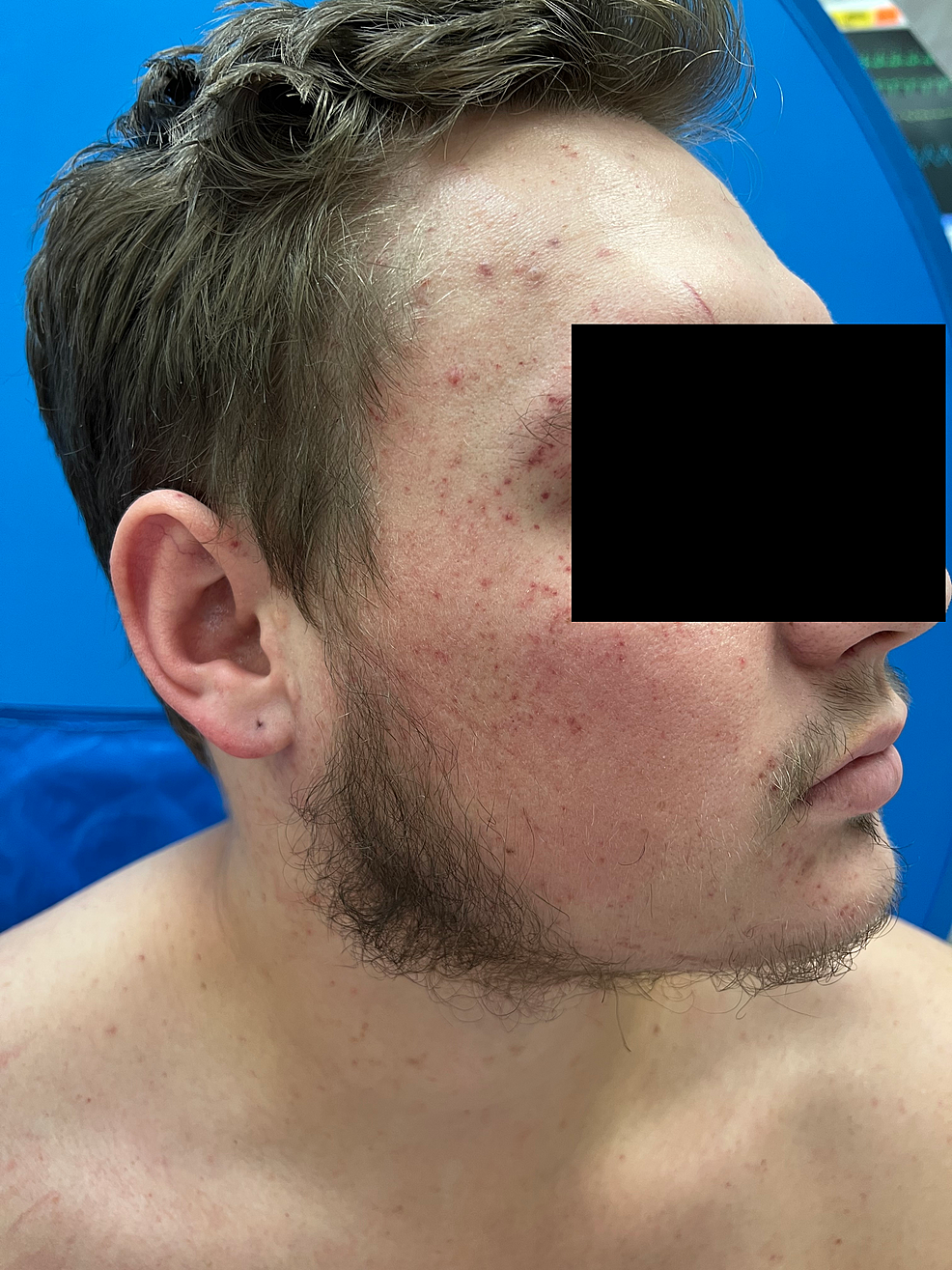The image shows a detailed side profile of a young Caucasian man in his 20s, who is shirtless and looking to the right. His eyes, upper nose, and eyebrows are obscured by a black rectangle, concealing his identity. He has medium-length, wavy brown hair, with a prominent hairstyle featuring thick sideburns and a patchy beard. Sparse facial hair includes a faint mustache, scruff under his chin, and a slight goatee. His face is marked with considerable acne, particularly around his forehead, cheeks, and eyes, indicating possible inflammation or minor injuries.

His right ear appears pierced, although there’s no earring present. In the background, a striking blue color dominates, possibly hinting at a swimming pool or a medical environment like a doctor’s office, and there may be indistinct green and yellow objects further back. The context, slightly suggested by one of the captions, may imply a hospital setting, possibly a waiting room or clinic, but this is not confirmed. The image captures an honest and raw portrayal of the man's physical appearance.